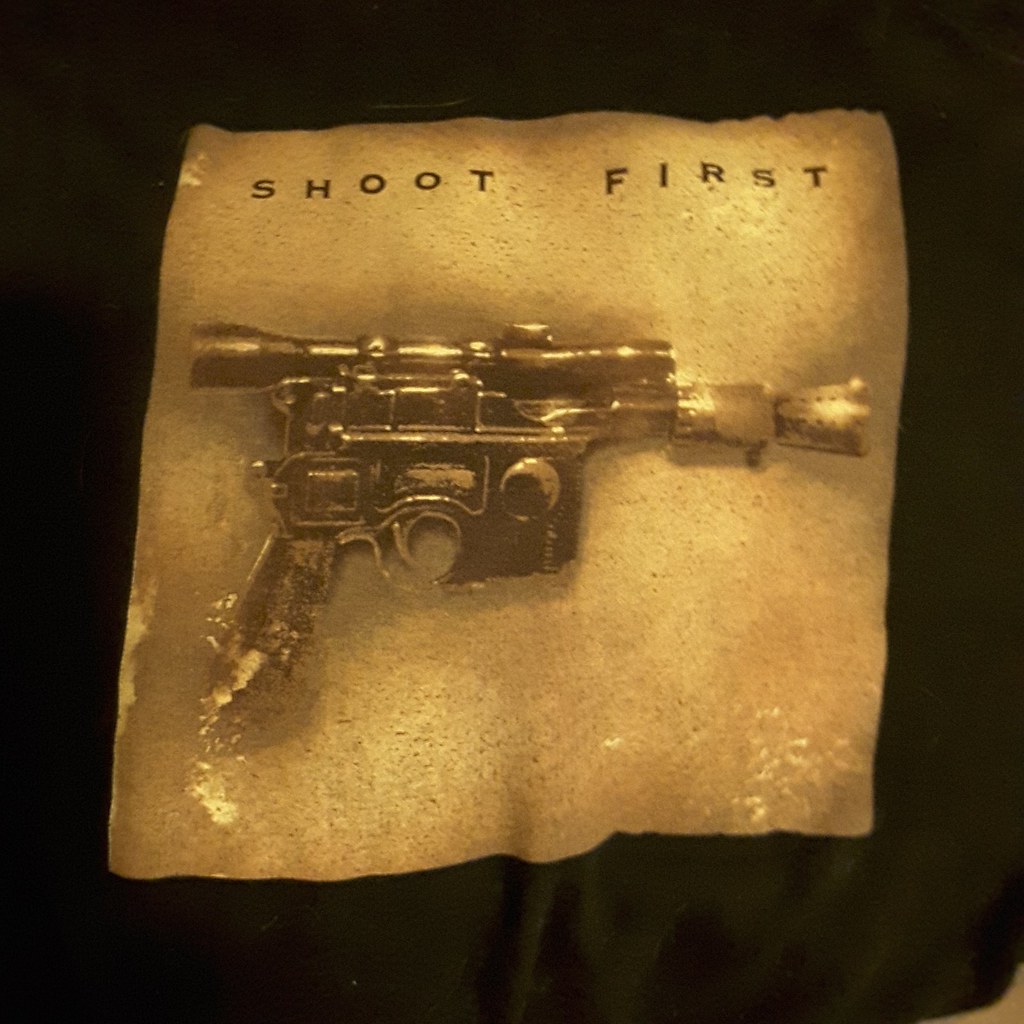This image depicts an antique-looking small handgun with a scope, seemingly inspired by a vintage or steampunk aesthetic, printed on a black fabric, likely a t-shirt. The print mimics the appearance of an old, yellowish-brown, worn piece of paper with a burnt effect around the edges. The handgun, which has a glossy and reflective finish, suggests a design from the 1950s or 1960s, filled with intricate, old-style contraptions. At the top of the image, in thin black capital letters, the text "SHOOT FIRST" is prominently displayed, possibly indicating a warning or gun advocacy message. The overall black and white design of the gun adds to the vintage and aged feel of the image.